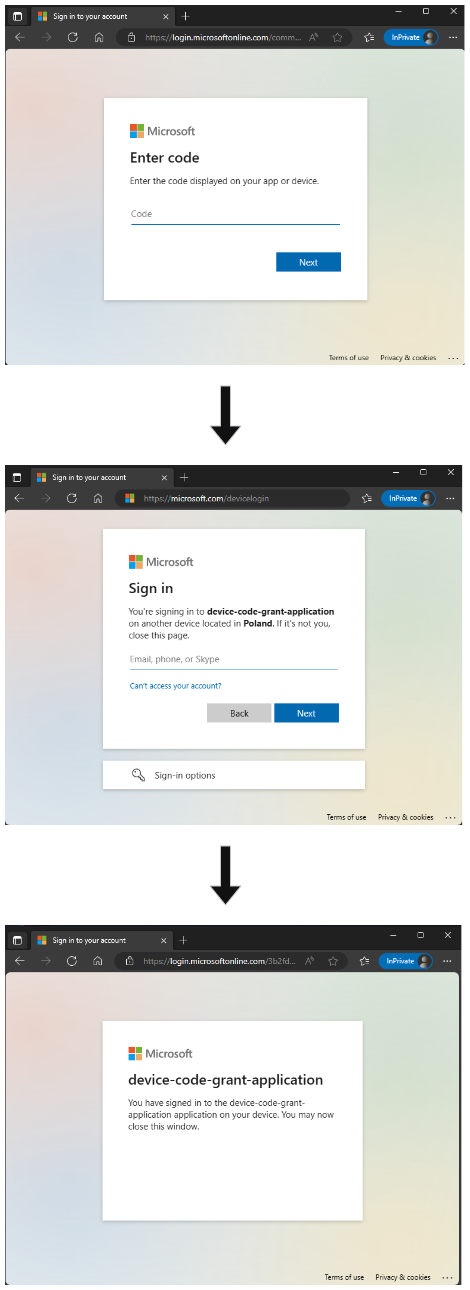The image features three sequential screenshots that detail the Microsoft login process, presented within a dark mode browser interface. Each screenshot is encapsulated within a white box set against a blurred, multicolored background incorporating shades of red, green, yellow, and blue.

At the top of each box, the Microsoft logo is prominently displayed, establishing the authentication context. Below the logo, the first screenshot is labeled "Enter Code" and instructs users to input the verification code shown on their app or device. A blue input field is provided for entering the code, along with a blue "Next" button at the bottom.

The second screenshot is labeled "Sign In," featuring a field to enter the user's email address. Arrows guide the viewer's attention from one step to the next, clearly delineating the login steps.

This detailed, step-by-step guide is visually organized to facilitate users in completing the Microsoft login process efficiently.